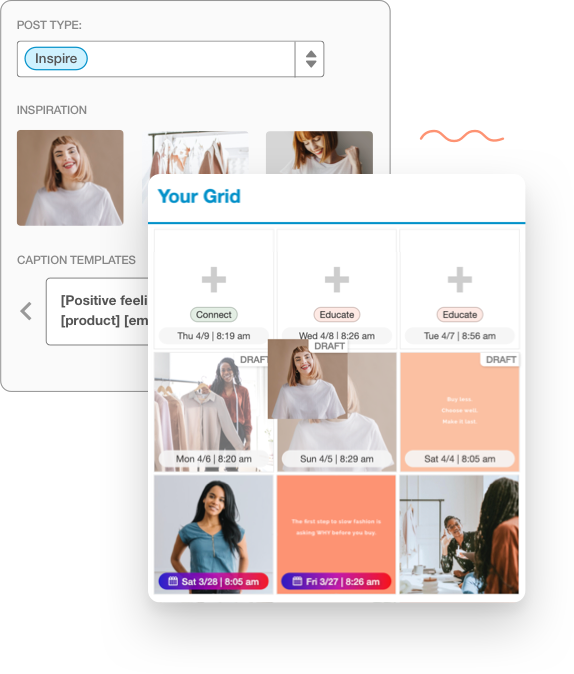The image depicts a digital layout featuring various elements arranged in a grid format. There are two main vertical rectangle sections. The lower rectangle, situated at the bottom left, has another rectangle overlaid on its bottom right corner.

The rectangle on the bottom left contains the text "Post Type: Inspire" followed by "Inspiration." Below this text, there are three photographs in a row. Under these photos, it reads "Caption Template: Positive Feeling Product."

The overlaid rectangle on the top left has the phrase "Your Grid" in blue text, accompanied by a blue line. This section is divided into a grid containing nine boxes, with three rows of three boxes each.

- The top row of boxes is empty, each displaying a gray plus sign and the text "Connect Thursday 4/9 8:19 AM."
- The second row of boxes is labeled "Educate" with respective dates and times: "Wednesday 4/8 8:24 AM" for the first box, "Wednesday 4/8 8:26 AM" for the second, and "Tuesday 4/7 8:56 AM" for the third, all including the gray plus sign.
- The third row contains drafted posts, labeled "Draft" with respective dates and times: "Monday 4/6 8:20 AM," "Sunday 4/5 8:29 AM," and "Saturday 4/4 8:05 AM."

Each box, either labeled or empty, maintains a white background with gray plus signs to indicate areas where content can be added.